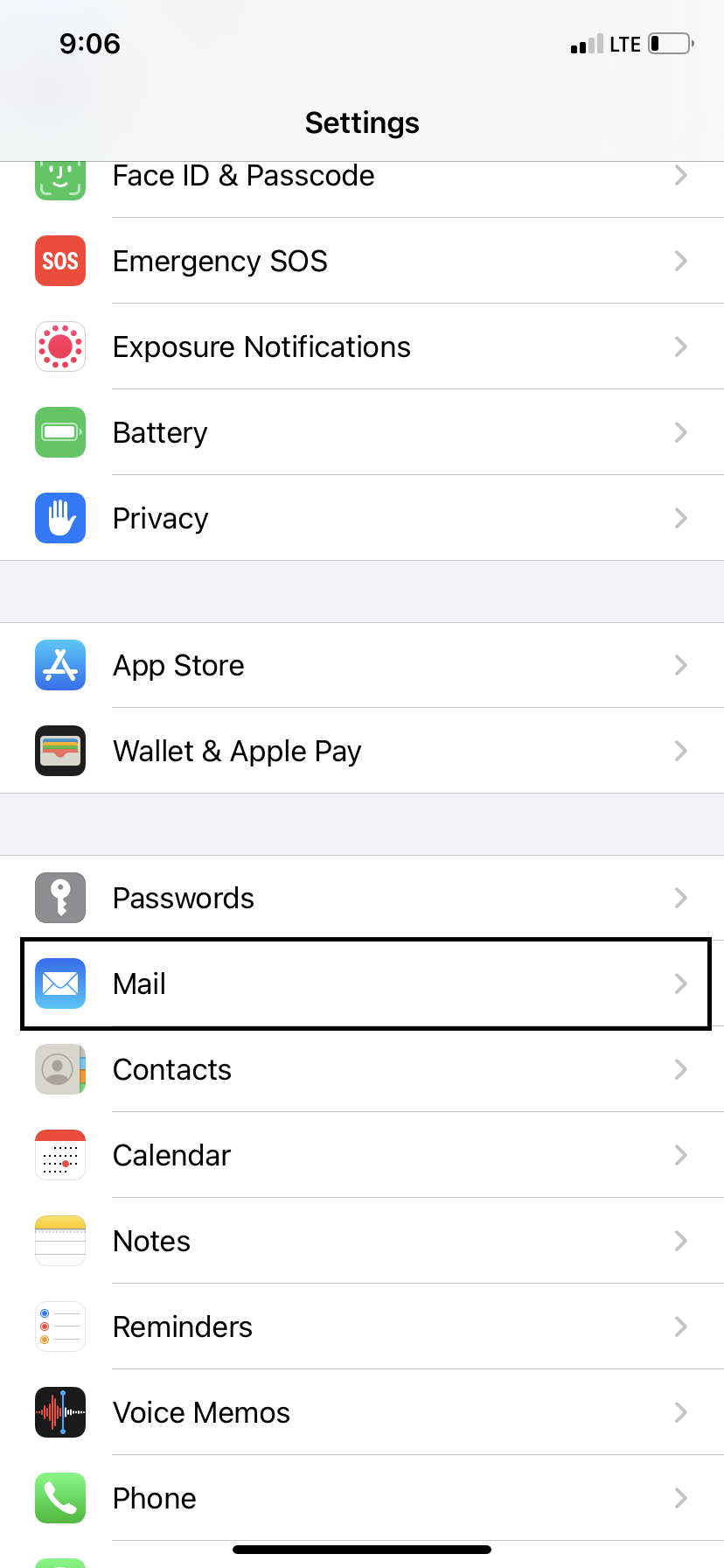This is a detailed description of a screenshot from a smartphone's settings page. The top of the screen features a gray status bar. On the left side of the bar, it displays the number "906" in bold font. On the right side, it shows a signal indicator with two out of four bars illuminated, the LTE label, and a nearly depleted battery icon. At the bottom center of the screen, the word "settings" is displayed.

The settings page is divided into categories, each separated by thick dove gray lines. 

- **First Category:**
  - **Face ID & Passcode:** Represented by a green icon.
  - **Emergency SOS:** Indicated by a red square icon with "SOS" in white font.
  - **Exposure Notifications:** Depicted with a white square featuring a red sun icon.
  - **Battery:** Displayed with a green square containing a white battery icon.
  - **Privacy:** Shown with a blue square that includes a hand icon. 
  - All these items have right-pointing arrows on their right end.

- **Second Category:**
  - **App Store:** Symbolized by a blue square with an "A" inside.
  - **Wallet & Apple Pay:** Represented by a black square with a credit card portfolio icon.

- **Final Category:**
  - **Passwords:** Presented with a gray box featuring a key icon.
  - **Mail:** Highlighted as selected, with a black box surrounding the app, depicted by a blue square containing a white envelope icon.
  - **Contacts:** Shown with a gray square that includes a circle with a head and shoulders inside.
  - **Calendar:** Displayed with a white square containing dots, one of which is marked with a red dot.
  - **Notes:** Represented by a white square with lines.
  - **Reminders:** Depicted with a white square that has colored dots (blue, red, and yellow) on the left side followed by gray lines.
  - **Voice Memos:** Shown with a black square featuring sound waves.
  - **Phone:** Displayed with a green square containing a white handset icon.